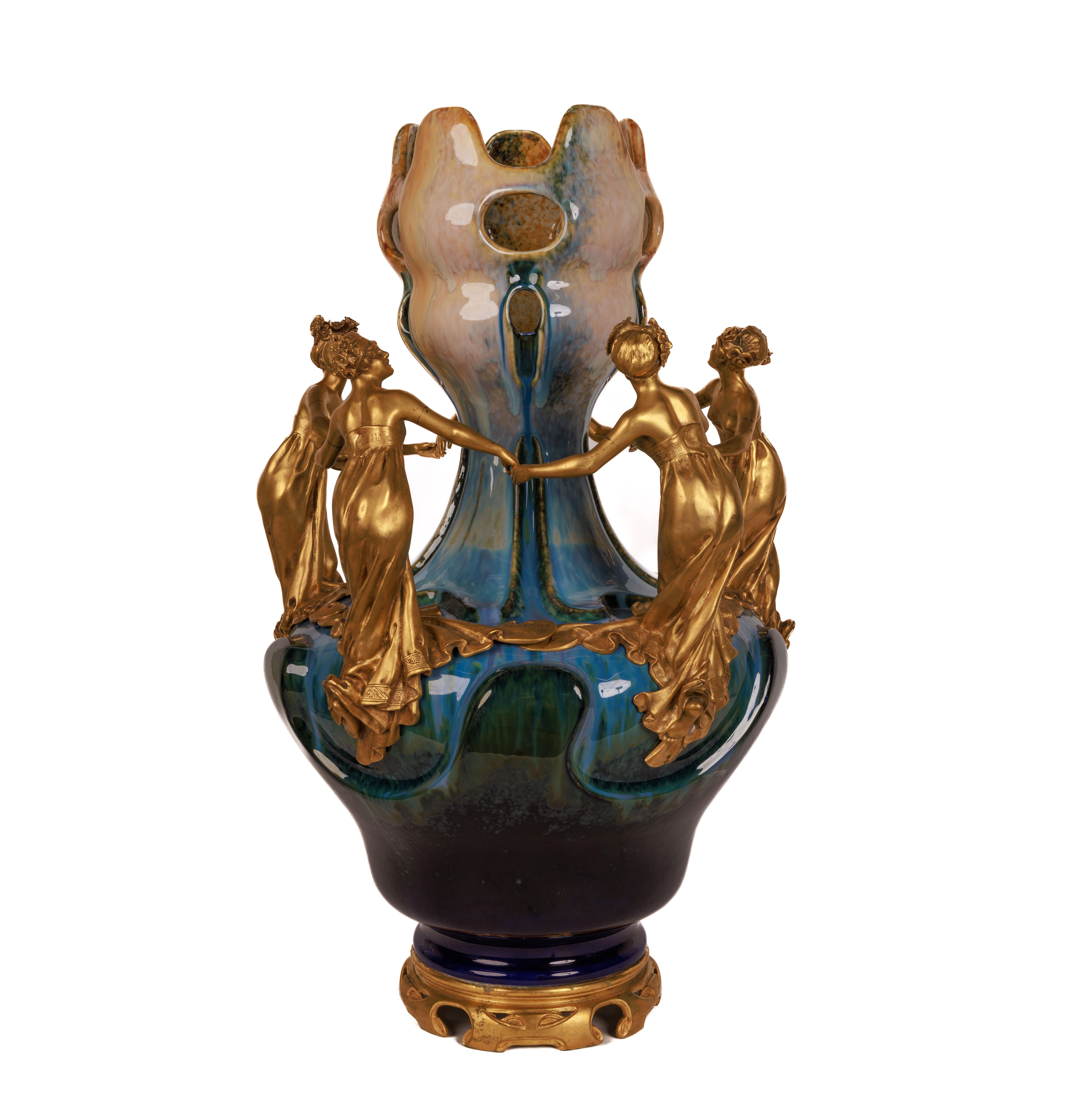The image depicts a unique and elaborate piece of pottery, possibly a vase, characterized by its striking design and vibrant colors. The vase is seated on a golden pedestal and features a high gloss glaze. The base of the vase starts with a deep, navy blue that gradually transitions into a lighter hue as it ascends. The vase flares out in the middle, narrows significantly, and then widens again towards the top which culminates in a beige color. Around the narrow center, four women, resembling Greek goddesses, are sculpted in flowing, golden gowns and are depicted holding hands. Their presence adds to the vase's intricate detail, giving it a sense of unity and grace as if they are engaged in a ritual dance or chant. The top portion of the vase, which subtly opens like a clam, showcases a spectrum of colors from light blue, peach, tan to brown, resembling stained glass with several holes cut into it. The women, the color gradient, and the detailed craftsmanship suggest that this pottery piece is not just functional, but also an exquisite piece of art.